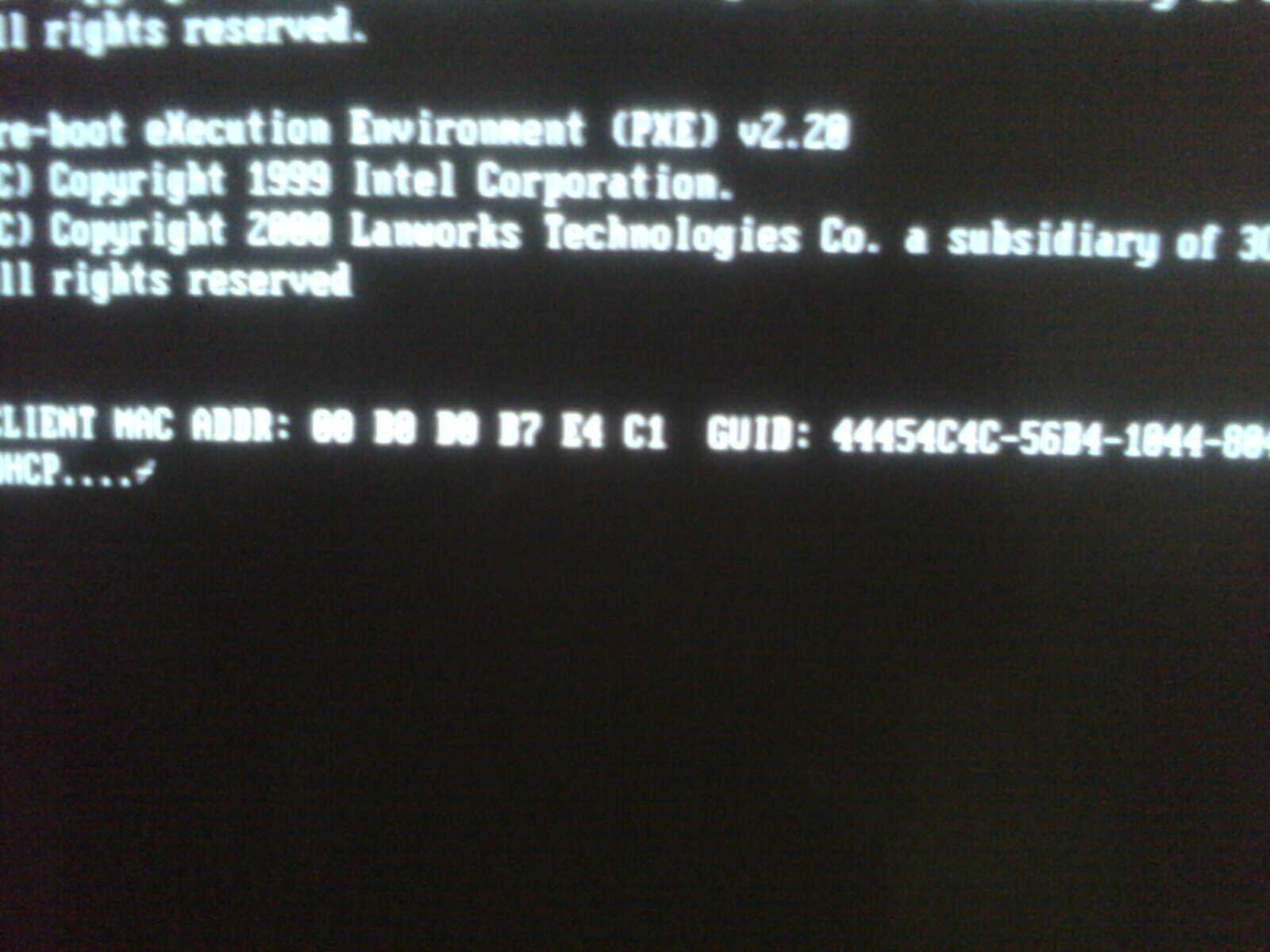The image depicts a classic computer boot screen with a black background and intensely bright white text, giving it a somewhat blurry appearance due to the high contrast. The screen features approximately six to seven rows of partially visible sentences, starting with a cut-off letter "L" followed by "Writes, Reserved." The text then has an indentation and begins with "RE-BOOT EXECUTION ENVIRONMENT (PXE V2.20)," followed by "copyright 1999 Intel Corporation, copyright 2000 Landworks Technology Company, a subsidiary of 3," before being abruptly cut off. Phrases like "All writes reserved," appear twice, although slightly cut off, especially affecting the letter "A." The majority of the text is in capital letters, including proper names, and includes a mix of technical terminology and standard phrases common in pre-boot environments for older computers.